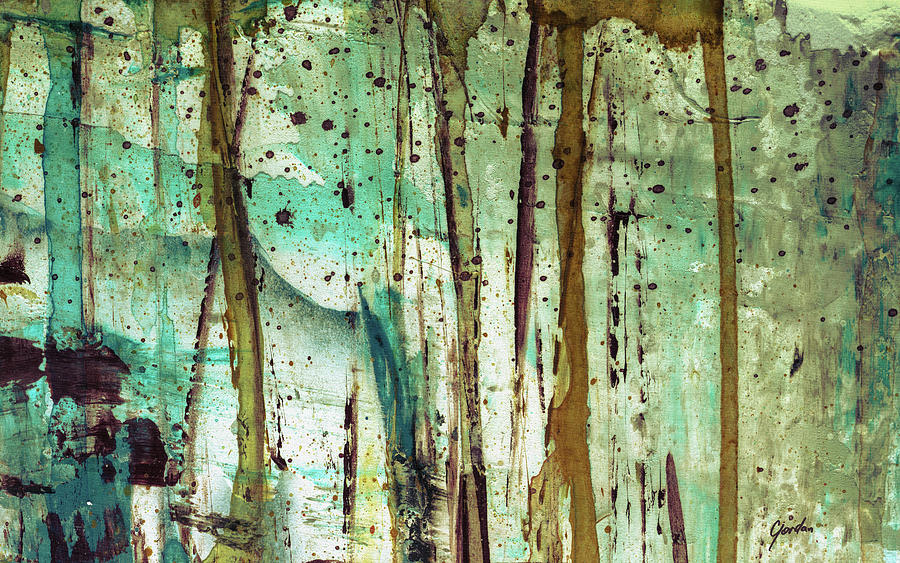The image is an impressionist-style watercolor painting primarily featuring shades of blue, white, brown, and light blue, with an overall color palette that includes muted tones such as turquoise and aquamarine, contrasted by dun shades of brown. The darker shades of blue and brown are predominantly seen, with black dots scattered throughout the composition. There are various stylistic elements including sweeping arches, waves, and dripping streaks. The brown paint appears to be applied at the top and allowed to drip down the canvas, adding a vertical motion to the piece. 

The lower right corner features a dark blue hue with a couple of black splotches, while light blue seems to act as a background, overlaid with white. Towards the left-hand side, the painting takes on a grayish-white tone. Despite its abstract presentation, the artwork evokes an impression of trees in a forest, with the brown streaks suggestive of tree trunks. Additionally, the painting does not have bright highlights and seems to be layered in its construction, suggesting a deliberate and thoughtful application of paint, likely done with acrylics. The painting is signed "Gordon" in the lower right corner.